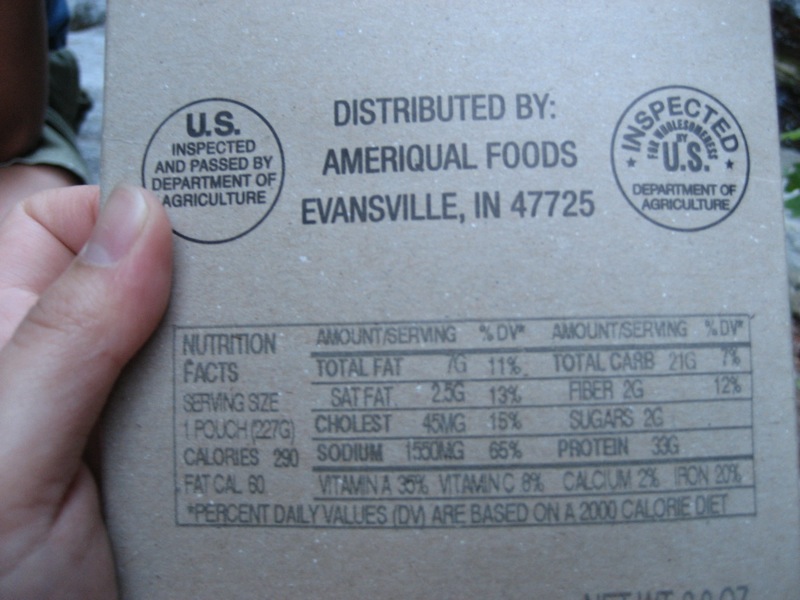In this vibrant color photograph, a human hand prominently displays a product label. The hand is clearly visible, with the thumb and forefinger delicately gripping the label, providing a sense of scale and interaction. To the left of the hand, another individual is partially visible, identifiable by the sleeve and an arm, suggesting a casual, possibly collaborative setting.

The label itself is stark white, accentuated by neat, black handwriting. On the left side of the label, a circular seal reads, "U.S. Inspected and Passed by Department of Agriculture." This assurance of quality and safety stands out and draws attention. 

Central to the label are several lines of text in all capital letters, crisply stating, "DISTRIBUTED BY AMERICORPS FOODS, EVANSVILLE, INDIANA, 47725." This central block of text provides key distribution information, ensuring clarity and authenticity.

On the right side of the label, another circular seal mirrors the left, reaffirming, "INSPECTED FOR [specific details obscured] U.S. Department of Agriculture," doubling down on the product's compliance and verification.

Below this, the nutritional information section is laid out methodically, offering detailed insights into the contents, including calorie count and other vital nutritional facts, making it easy for consumers to make informed choices.

Overall, the photograph is a detailed and reassuring display of product information and inspection, highlighting both human interaction and regulatory assurance.